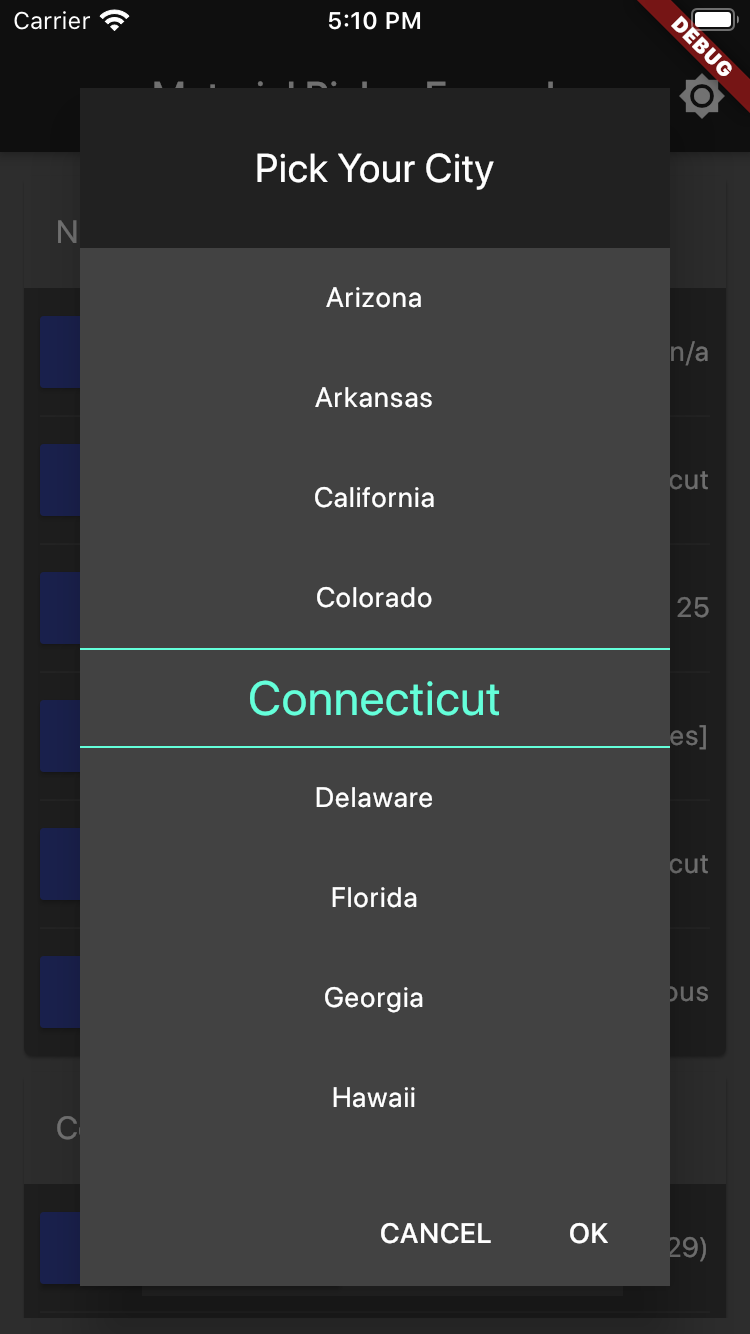The image, taken from a smartphone, is presented in a vertical format, primarily featuring a dark background of varying shades of black and dark gray. At the top left corner, the word "carrier" appears in white text alongside a Wi-Fi icon. Centrally positioned is the time, displayed as "5:10 PM." In the upper right corner, there is a battery life icon with a "debug" strip superimposed on it.

The focal point of the image is a gray pop-up box titled "Pick Your City" in white text. Below the title, several state names are listed in white against the gray background, starting with "Arizona," "Arkansas," "California," and "Colorado." A seafoam green line separates these names from "Connecticut," which is displayed in a larger font and in the same color. Another green line follows, segmenting "Connecticut" from the subsequent list of states: "Delaware," "Florida," "Georgia," and "Hawaii."

At the bottom of the pop-up box, there are two buttons in uppercase white text reading "CANCEL" and "OK." This gray pop-up box overlays an obscured background featuring hints of blue boxes with white text, details of which are not discernible due to the overlay.